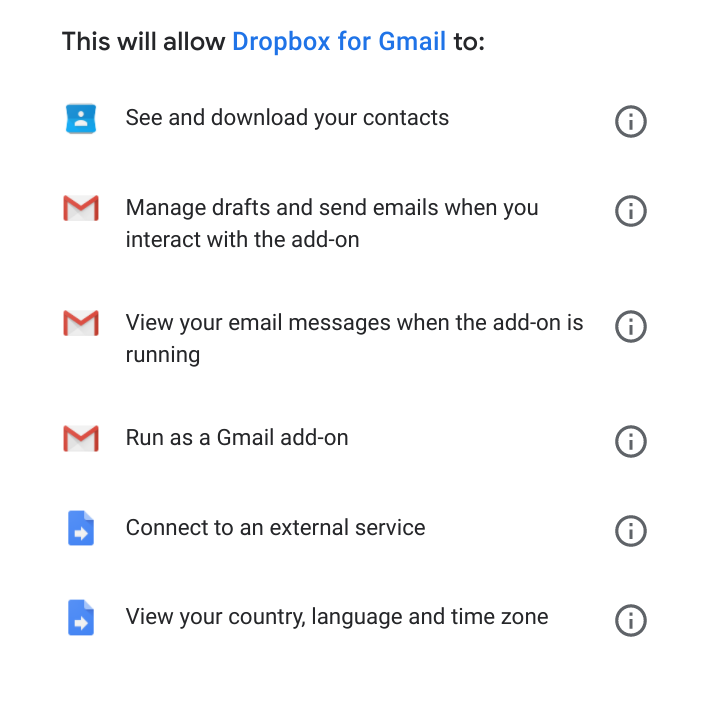The photo depicts a screen showcasing the setup stage or settings for the product "Dropbox for Gmail." The screen details the permissions required for this add-on, including the ability to: 

1. Access and download your contacts.
2. Manage drafts and send emails when you interact with the add-on.
3. View your email messages while the add-on is active.
4. Function as a Gmail add-on.
5. Connect to an external service.
6. View your country, language, and time zone.

Each permission is accompanied by a small icon of the letter "i" within a circle, which users can click for more information and detailed descriptions to understand the implications of the permissions. This setup screen essentially informs users of the actions and data the add-on will have access to if they choose to install it.